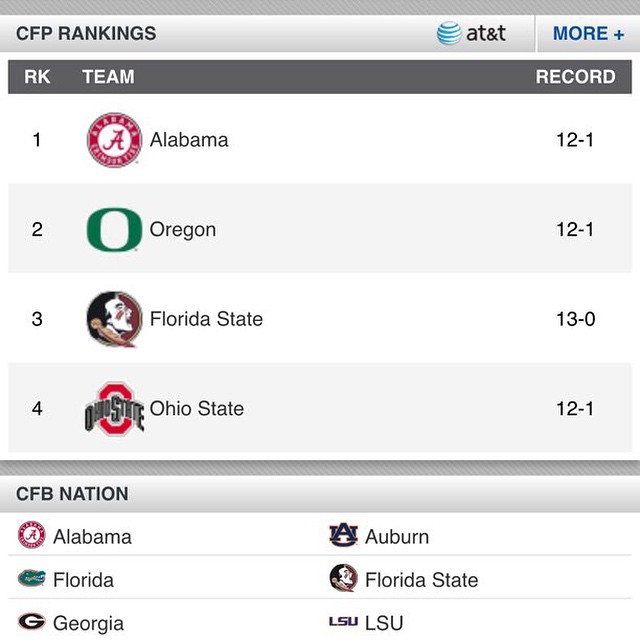This image appears to be a screenshot of a mobile website displaying sports rankings, specifically the College Football Playoff (CFP) rankings. The screen is primarily light and dark gray, featuring a prominent header at the top that reads "CFP Rankings" in bold black letters. In the upper left corner, there's an AT&T logo with blue stripes accompanied by the text "MORE+."

Below the header, a table lists the top four teams with their respective ranks, team names, records, and logos: 
1. Alabama (Record: 12-1) – represented by a red circle with a white 'A' in the center.
2. Oregon (Record: 12-1) – represented by a green 'O'.
3. Florida State (Record: 13-0) – represented by a logo depicting a screaming Native American with a feather in his hair.
4. Ohio State (Record: 12-1) – represented by a red 'O' with the text "Ohio State" in curved letters around it.

Below this table, there is another section titled "CFB Nation" set against a band of gray. This section lists six additional teams, split into two columns. The left column lists Alabama, Florida, and Georgia, while the right column lists Auburn, Florida State, and LSU, each with their respective logos next to the team names.